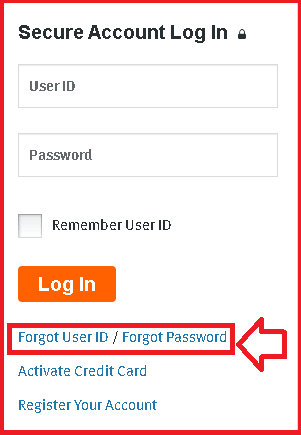The image appears to be a low-resolution screenshot of an instruction page, focused on guiding users through the account login and recovery process. The entire image is surrounded by a red border and features a white background. 

At the top, there is bold black text that reads "Secure Account Login" accompanied by a lock icon to its right. Below this are two input fields with grey outlines: the first one labeled "User ID" and the second labeled "Password." 

Below the password field, there is an unchecked checkbox next to the text "Remember User ID." Further down, an orange button with white text reads "Login."

Underneath the login button, there are three links:
1. "Forgot User ID / Forgot Password" – highlighted by a red box around it and a red arrow pointing towards it from the right.
2. "Activate Credit Card."
3. "Register Your Account."

The image suggests instructional content primarily focused on helping users retrieve their forgotten user ID or password.